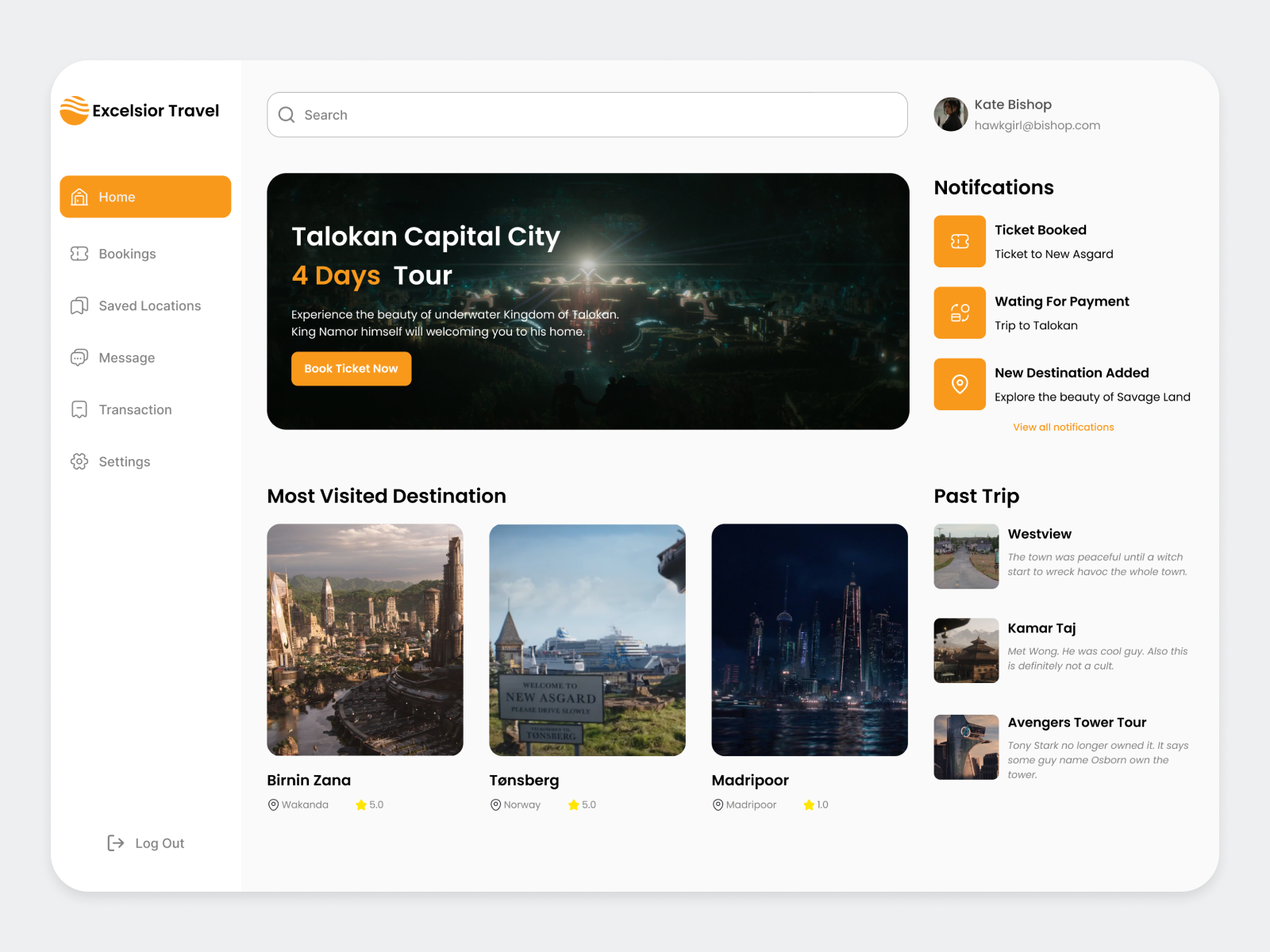**Excelsior Travel Dashboard**

The image features a clean, white background with the Excelsior Travel page header prominently displayed in the top-left corner. The Excelsior Travel icon is a vibrant orange circle featuring three horizontal white lines in its upper portion. Positioned at the top center is a functional search bar, while the top right corner displays the user's email address, katebishophawkgirlatbishop.com, accompanied by a notification panel.

The notification panel contains various alerts, each marked with an orange icon:
- **Ticket Booked**: Confirmation of a ticket to New Asgard.
- **Pending Payment**: A pending payment for a trip to Tolocan, represented by an orange coin icon.
- **New Destination Added**: An announcement of a new destination, Surfer's Ledge, with an orange location pin icon.

At the bottom of the notification panel, there is an "View All Notifications" button highlighted in orange, followed by a section titled "Past Trips". Here, users can reminisce about previous adventures:
- **West View**: "The town was peaceful until a witch started to wreak havoc."
- **Karma Touch**: "Met Wong, a cool guy, definitely not a cult."
- **Avengers Tower**: "Some guy named Osbourne owns the tower now."

On the right side of the page, a vertical side menu lists navigation options, with "Home" highlighted in orange. Other options include:
- Booking
- Save Location
- Messages
- Transactions
- Settings

The central portion of the image showcases a travel highlight: "Tolocan Capital City - 4 Days Tour." The '4 days' text is prominently colored in orange. The description reads: "Experience the beauty of the underwater kingdom of Tolocan. King Namur himself will welcome you to his home." Below this text is a bright orange button labeled "Book Ticket Now."

Further down, the most visited destinations are listed, emphasizing popular travel spots:
- Benin Zana, Botswana
- Wakanda
- Tonsberg, Norway
- Madripoor (listed twice, likely an error or a visual emphasis on this destination).

This descriptive caption provides a detailed overview of the various components and features depicted in the image, ensuring clarity and engagement for the reader.